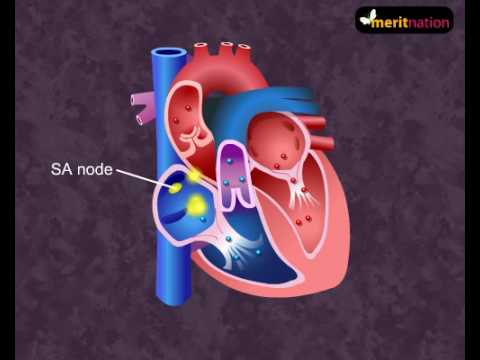This detailed illustration depicts a cutaway view of the heart, focusing on its internal structure and key components. The image, which features both red and blue sections to differentiate various heart compartments, showcases four distinct chambers. A large blue vein traverses the left side of the heart, while the main muscle mass occupies the right. 

Notably, small blue and red dots appear within each chamber, illustrating blood flow. The SA Node, critical for heart rhythm, is highlighted with yellow circles and a labeling line pointing to it; it's situated in the upper part of the heart and distinctly marked as "SA Node" against a dark gray background. The node is depicted as resembling a jellyfish with floating yellow bits within a blue segment.

This educational illustration is branded with "Merit Nation" at the very top right corner, set against a small black area. The overall image has a dark gray backdrop, complemented by a thick black border on both the left and right sides, enhancing the heart's vivid colors.